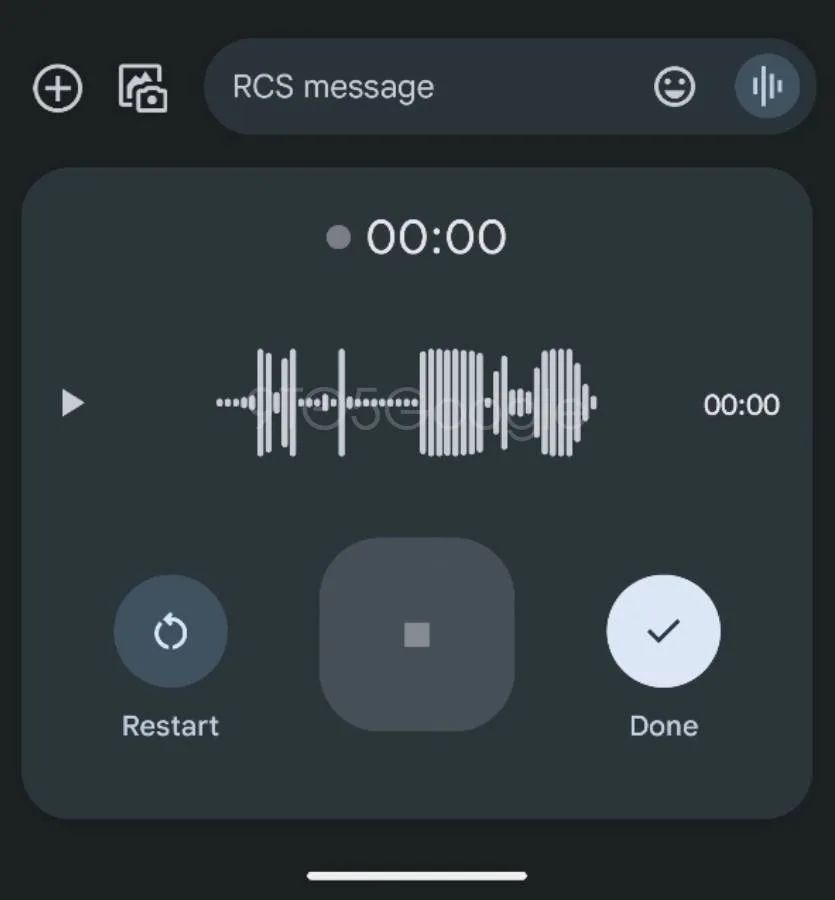The image displays an RCS (Rich Communication Services) message interface set against a black background. The screen features a mixture of white and gray text. Dominantly visible is a voice recorder interface, complete with a play button prominently centered on the screen. Surrounding the play button are additional controls: a restart circular button and a stop button, the latter rendered in a lighter gray. A "Done" button is clearly visible, marked by a white check mark within a gray circle. To the right of these controls, white lines trace the waveform of recorded audio, undulating to represent the voice modulation and pauses. A gray dot precedes the timestamp showing "00:00," indicating the recording's start. Overall, the interface is meticulously organized, with each element contributing to a coherent and user-friendly design.